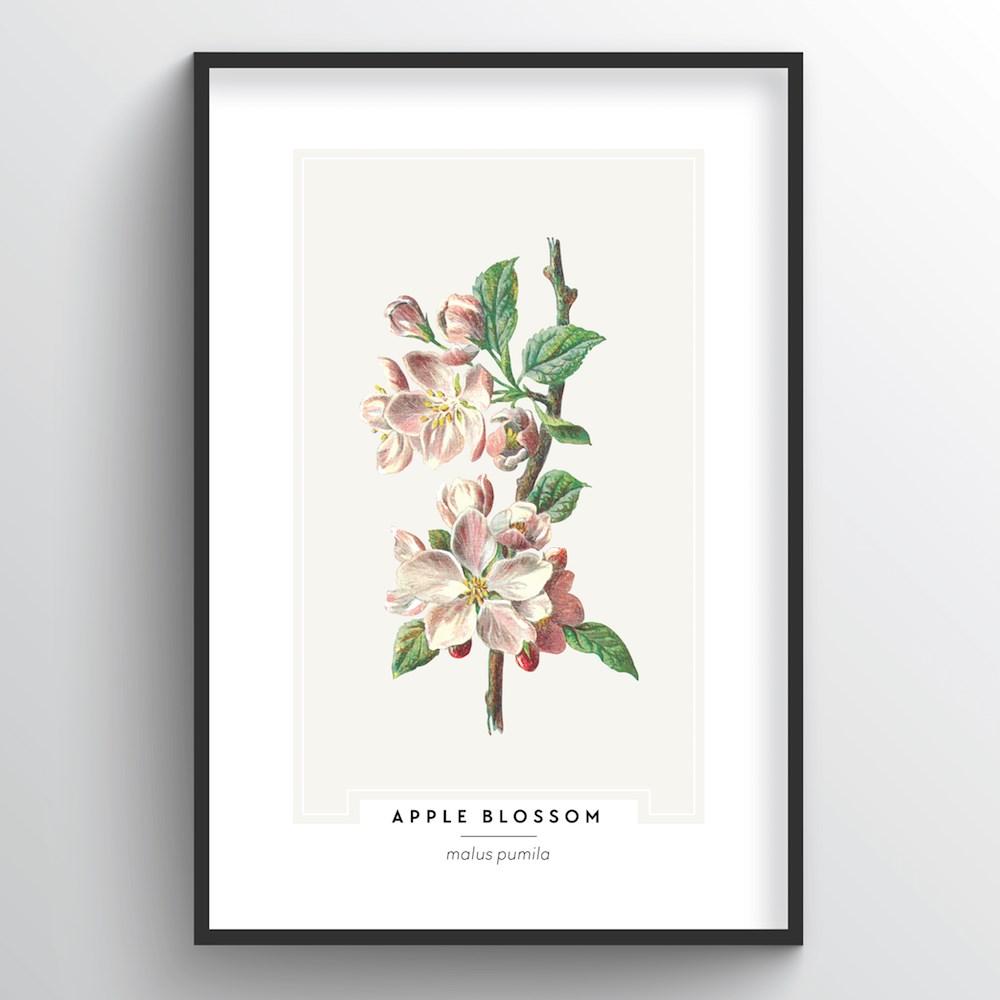The image is a detailed photograph of a framed piece of art hanging on a light gray wall. The artwork is presented in a sleek, thin black rectangular frame which encloses a wide white mat, adding depth and focus to the central subject. The art itself is a meticulously crafted painting or pencil drawing featuring a vertical apple blossom branch. The branch is adorned with green leaves, pinkish-white flowers, and small red buds, capturing the delicate beauty of apple blossoms. At the bottom of the artwork, in bold black uppercase letters, it reads "APPLE BLOSSOM," with a beige horizontal line underneath. Below this line, the scientific name "MALUS PUMILA" is elegantly inscribed, contributing an educational element to the piece. The precise medium of the artwork remains ambiguous, though it is suggested to be either acrylic or pencil.